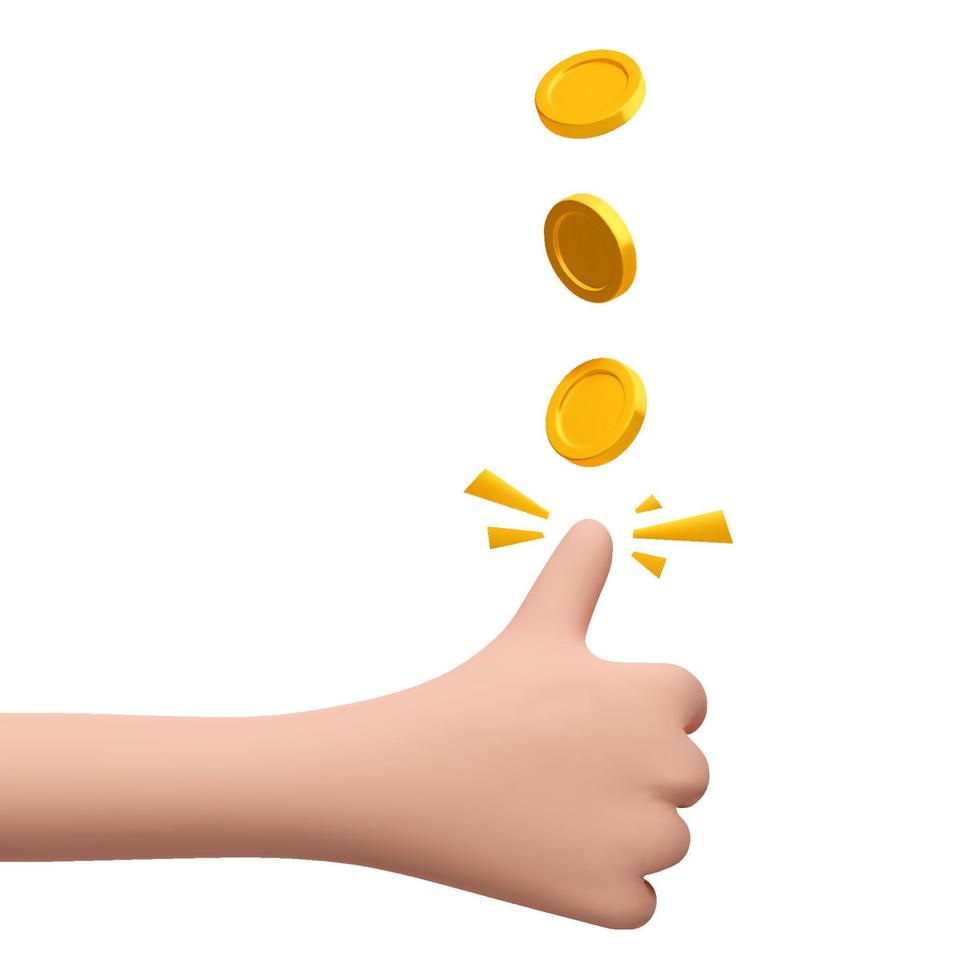This digital image features a section of a human arm, depicted from the mid-forearm down, with the hand prominently positioned against a minimalist white background. The hand's fingers are curled back towards the palm while the thumb extends straight up into the air. Surrounding the thumb are five small action lines or motion indicators, symbolizing the recent flipping motion. Hovering above the thumb are three small gold coins, captured mid-flip. The coins are positioned with the lowest one ascending towards the upper right corner, the middle coin angled towards the upper left, and the top coin remaining nearly horizontal. The image is void of any jewelry or additional adornment, emphasizing the dynamic motion of the thumb flipping the coins into the air.